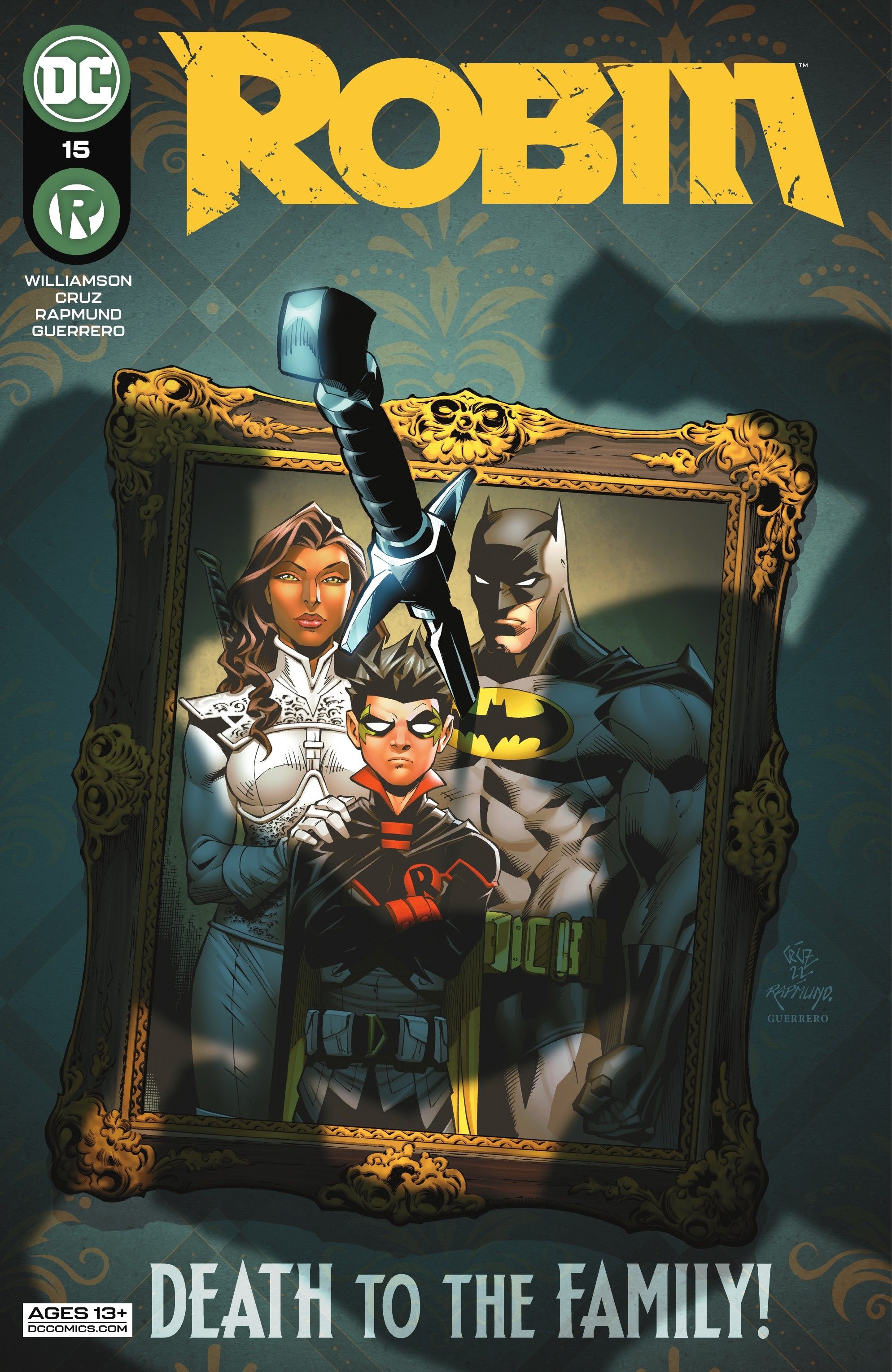This is the cover of a DC Comics issue. Dominating the top is the word "Robin" in bold yellow text, with the DC logo in a green circle to the left, and the number 15 below it. The background is a light blue with a subtle light gold floral pattern. A shadow of a fist is visible to the right. Below, a detailed portrait is framed in brown with gold edges. The portrait features Batman on the right, a woman on the left, and a child in a Robin costume in the center, with the woman touching the child's shoulder. A sword is dramatically stuck through the middle of Batman's chest. At the bottom, white text ominously declares, "Death to the Family." Additional details include the creators’ names — Williamson, Cruz, Ratmund, and Guerrero — and the note that the comic is suitable for ages 13 and up, with a reference to DCComics.com.